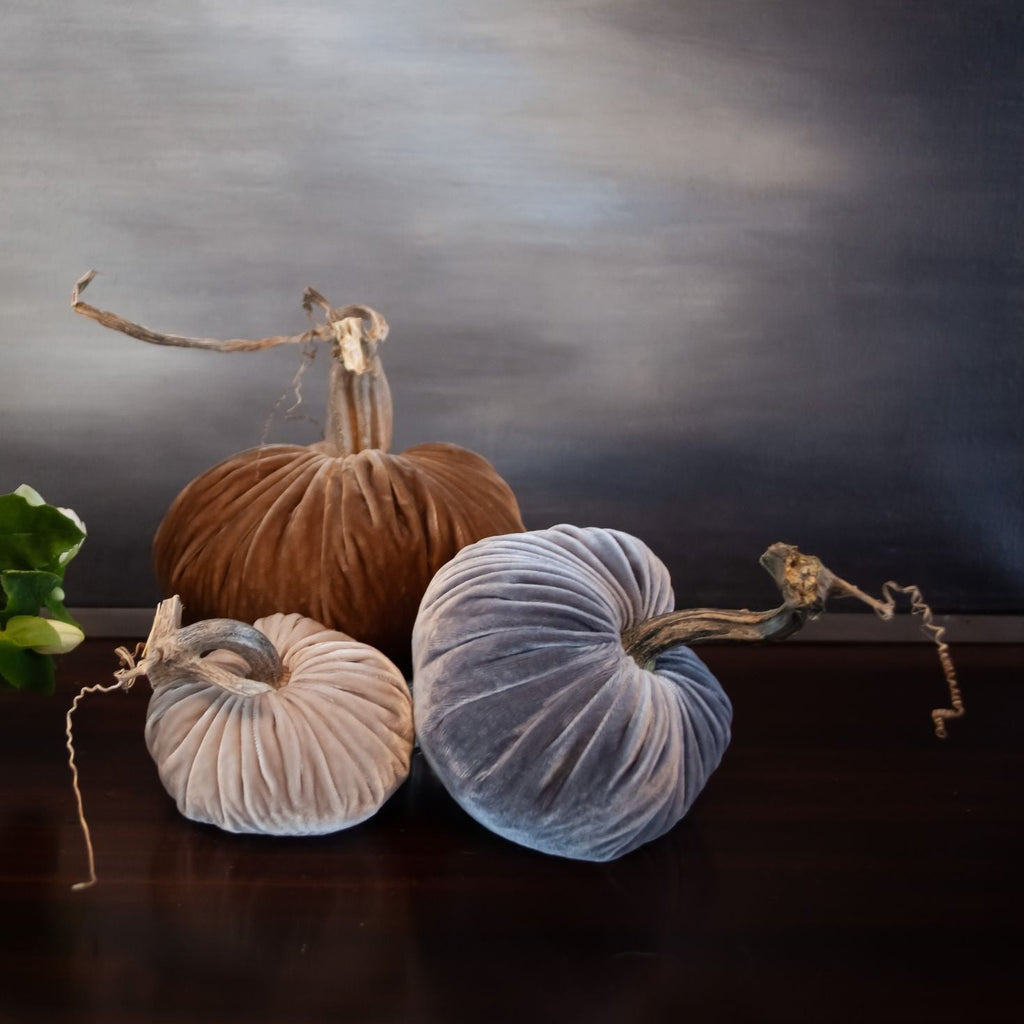This image, likely a painting or artistic print, features three fabric pumpkins set against a horizontally blended sky of gray, dark gray, and a touch of blue at the center, with a solid black surface at the bottom. The largest pumpkin is orange with a brown stem and is positioned in the center. To its left, a smaller white pumpkin with a curved brown stem is situated in the foreground. On the right, there is a blue and gray fabric pumpkin with a longer stem that tilts to the right. A few green leaves, dark with light lime accents, are visible towards the left side of the image.